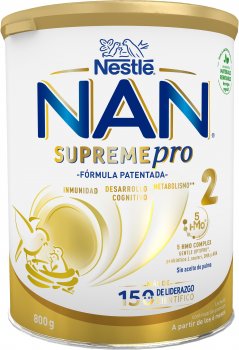This is a detailed product photograph of a Nestle Nan Supreme Pro canister. The can has a distinct gold top and a predominantly white body, accented by a gold band at the bottom. Central to the design is the Nestle logo at the top, which features an intricate illustration of a nest with a big bird feeding three smaller birds, accompanied by a butterfly. Immediately below this, in large, capitalized blue letters with a gold outline, is the brand name "NAN". The "NAN" lettering showcases a gradient effect with light blue transitioning into a darker blue, particularly the 'A' character which is entirely dark blue. Below "NAN", the words "Supreme Pro" are displayed; "Supreme" is in gold with an ombre effect and "Pro" is in blue, italicized font with a gold outline. Underneath, in smaller blue letters, is the phrase "Formula Patentada", indicating the patented formula in Spanish.

On the right-hand side of the can, there is a subtle image featuring a mother and child with a stork, symbolizing nurturing care. To the left, a prominent gold '2' marks the formula stage. At the bottom, the can indicates "150" years of Nestle's leadership in community development, metabolism, and cognition. Additionally, small text mentions "5-HMO", likely referring to a key ingredient, and states the canister's weight of 800 grams. The can's intricate design is further embellished by gold lines that start thick and then fade into thinner lines flanking the Nestle logo, adding to the premium aesthetic.